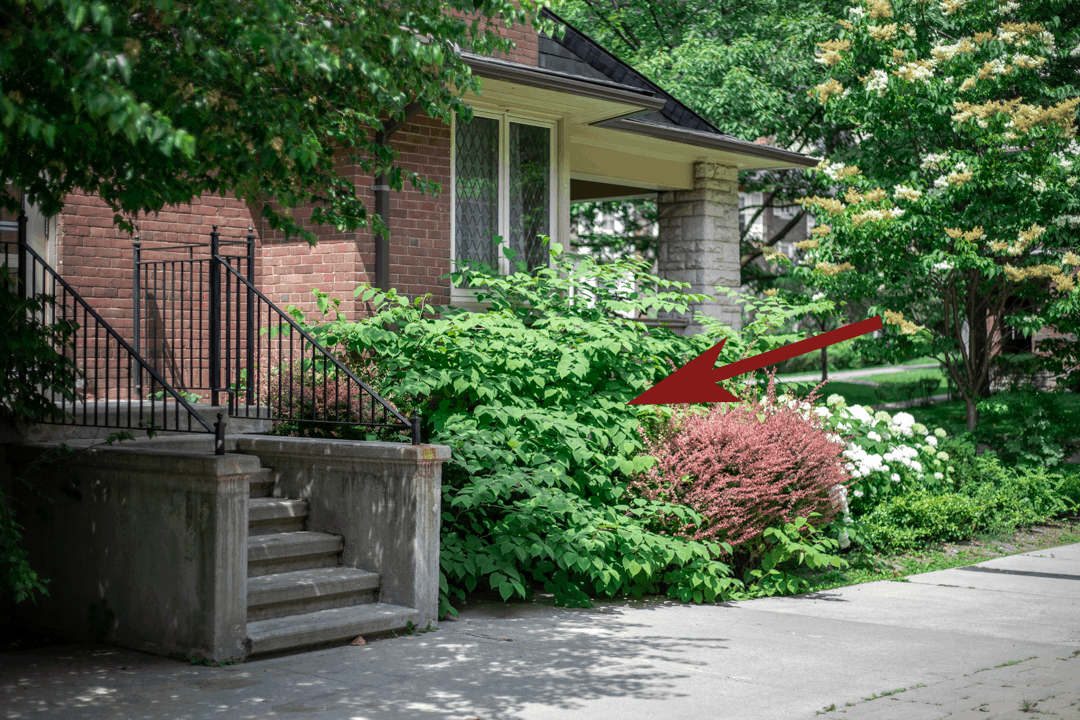This daytime photograph showcases the exterior of a red brick house. The house features a black shingled roof and a striking stone gray stanchion supporting the roof on the right. In front, concrete steps with a black metal handrail lead up to the entrance. On the left, two narrow windows punctuate the brick facade. The lush surroundings include various trees, some with green leaves and others adorned with white and light yellow buds. A garden at the front of the house boasts a vibrant red bush, numerous green plants, and clusters of white flowers. A conspicuous red arrow points towards the bushes in front of the house, indicating the area of the garden. The overall setting appears peaceful, adding to the house's charm in what seems to be a quiet and pleasant neighborhood.